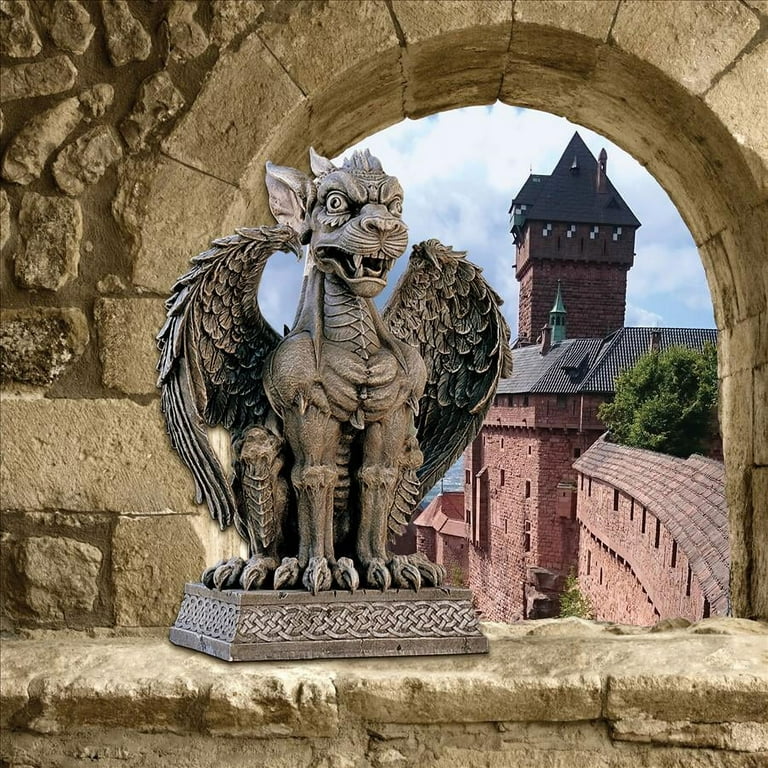This professional photograph captures a majestic greystone griffin statue positioned elegantly atop a ledge, peering out from an arched window of a castle. The background reveals the red walls and tower of another castle section. The arch is constructed from brick and cement, providing a rugged frame for the scene. Trees are visible atop a smaller roof on the right side, adding a touch of nature to the enchanting medieval setting. The griffin, a mythical creature, is depicted in a sitting position with its wings and ears pointed backwards. It has four legs with sharp claws, a menacing expression, bared teeth, and a slightly protruding tongue. The base of the statue is adorned with intricate Celtic symbols, enhancing its mystic allure.